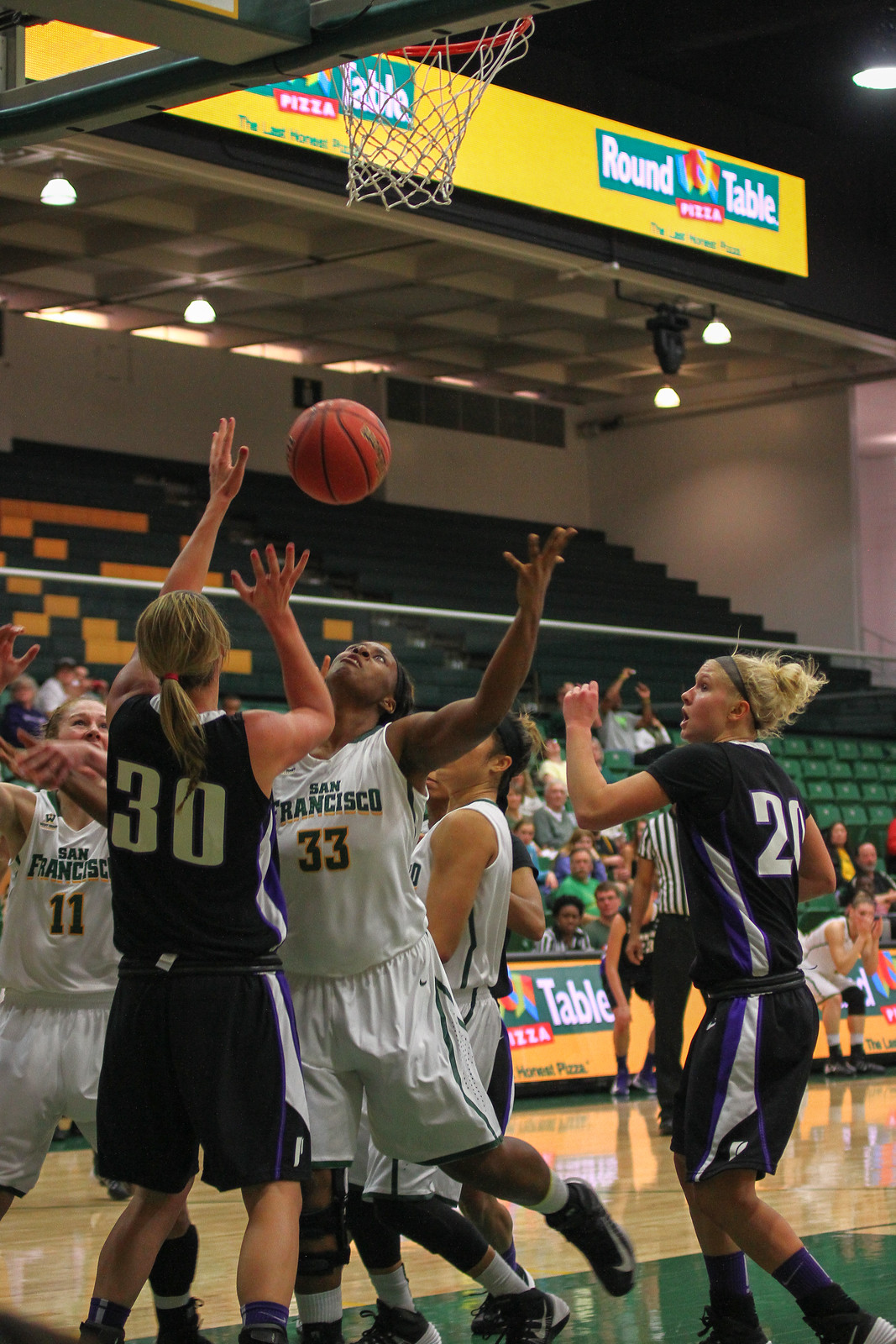The detailed photograph captures an engaging moment during an indoor girls' basketball game set in a well-lit stadium. The arena features white-painted walls and a striking vaulted ceiling in white and black. Hanging from the ceiling and prominently visible is a large yellow banner with a green rectangle reading "Round Table" in white font. The arena's seating area includes multiple levels of green and yellow chairs, which are partially populated with spectators, though the stands are not crowded.

In the foreground, a dynamic scene unfolds with players from two teams arrayed in purple and white jerseys—one marked with "San Francisco" and another with "Round Table Pizza." The players, numbering about seven or more, are clustered under the basketball net, vying for control of the ball, which is slightly left and above them. Additional elements, such as a scoreboard and a referee, are discernible in the background, alongside more spectators seated in the tiered stands.

The bottom portion of the image highlights the basketball court and hoop, while the upper section gives a full view of the audience area and additional large banners matching the one hanging above, reinforcing the "Round Table" theme. The detailed coloration includes white, green, black, purple, tan, and red accents, contributing to the lively and competitive atmosphere of the game.